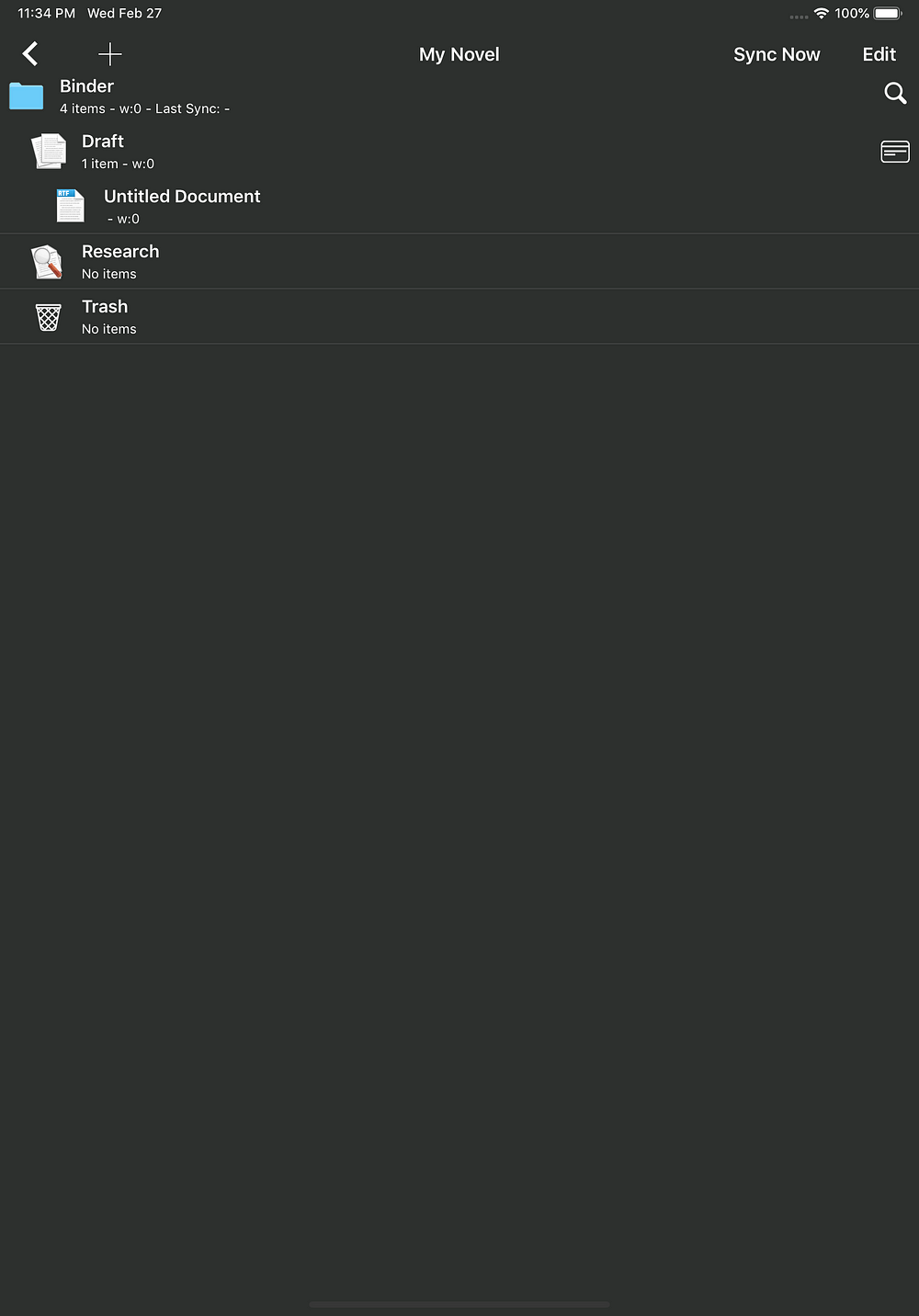The image depicts a digital workspace, likely an app or software used for writing novels. The main screen is predominantly black with centered white text that reads “My Novel.” In the upper right-hand corner, there's an "Edit" button. Directly above it, the battery meter indicates 100%, and the Wi-Fi signal is full. On the far left, there’s a timestamp showing 11:34 p.m., followed by the date, Wednesday, February 27th.

Beneath the title "My Novel" is an option labeled “Sync Now,” and an arrow to go back, with a "+" symbol beside it. Below this section, a tabbed blue folder icon labeled “Binder” appears. The binder lists four items, with each item name appearing in a smaller font size (approximately 10-point size) compared to the 14-point size of the main headings. 

Within the “Binder” section, there’s a subfolder marked with two paper document icons labeled “Draft” containing one item. Further indented, an untitled document is listed, also indicating one document with a small blue header. This document is also associated with a “Research” section, denoted by a magnifying glass icon over a piece of paper.

A "Trash" bin labeled “Trash” indicates no items within it. All elements are clustered towards the top, leaving about three-quarters of the screen blank and black, ensuring the user interface remains clean and organized. The font size varies to distinguish main headings from listed items, with the latter being smaller and unbolded.